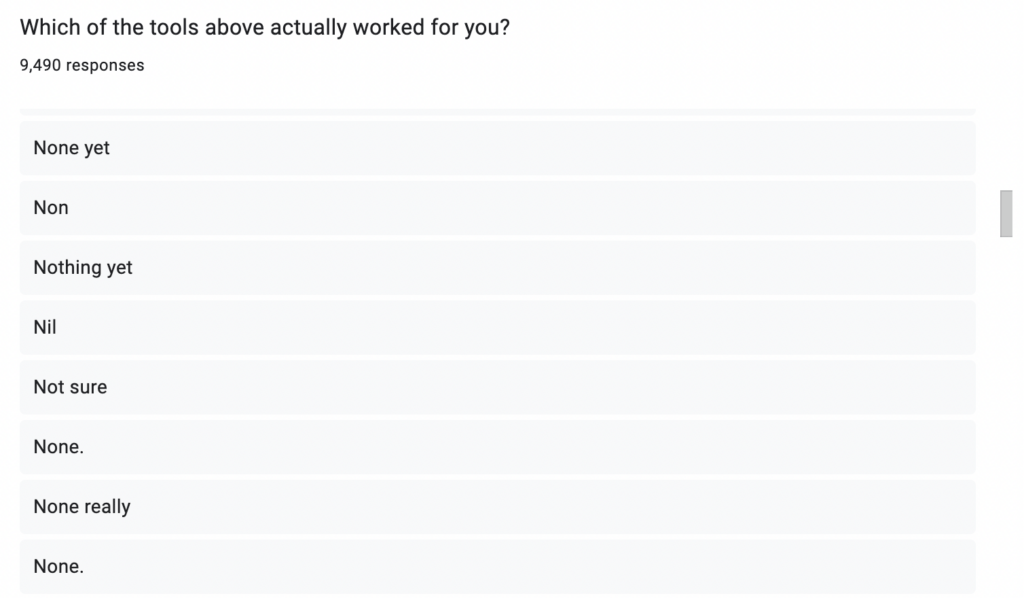The top left corner of the image displays a section titled "Which of the tools above have to work for you?" with 9,490 responses recorded. This section, along with a gray scrollbar on the right, is organized into 8 clearly defined subsections, each spaced apart from the others. The image highlights that, as of now, there seem to be no responses selected that indicate a preference for any of the tools listed.